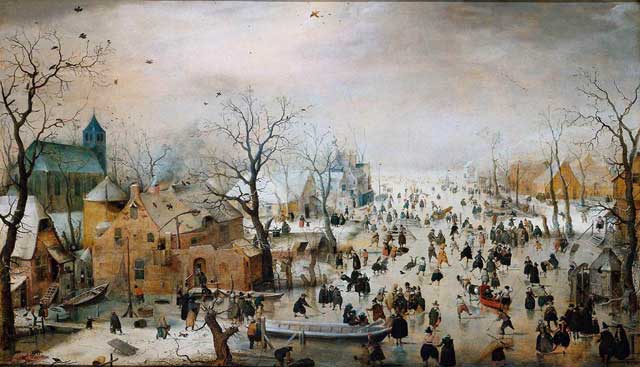This intricate artwork depicts an outdoor scene from an elevated perspective, showcasing the bustling square of a small village or town during the late fall or winter. The landscape is characterized by leafless trees, contributing to the season's chilly atmosphere. The sky, painted in white and brown tones, appears overcast and dreary, adding to the overall somber mood. A significant number of people are present, most dressed in dark clothing and indistinct due to their distance. They seem to be engaged in various activities, including skating on a frozen river, inferred from their postures and some holding hockey sticks.

Prominently in the foreground is an empty boat with oars sticking out, adding to the scene's narrative depth. On the left side stands a large house with a courtyard open to the icy river area, juxtaposed by a bluish-gray, church-like structure dominating the middle left background. Additional buildings painted in brown, blue, and white hues are scattered throughout, some possibly topped with snow, enhancing the wintry setting. Behind these buildings are smaller boats, indicating a riverside locale.

In the bottom right corner, a charming horse-drawn sleigh, painted red and carrying three or four people, adds a nostalgic touch. The painting is punctuated with elements evoking the era, such as people pushing sleds, cleaning streets, and building boats and structures, suggesting a busy day in a medieval or Victorian town. Despite the lack of facial details on the figures, their presence enlivens the scene, vividly capturing the essence of communal life in a bygone era. The overall effect is a richly detailed and atmospheric portrayal, reminiscent of scenes from a Charles Dickens novel.